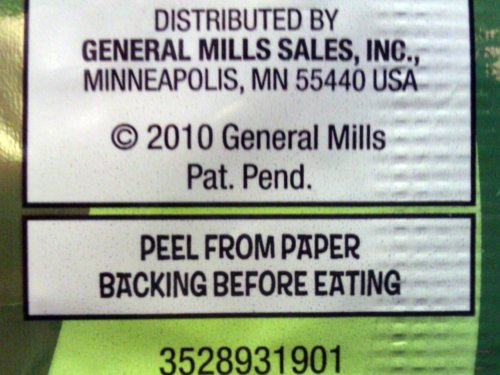**Caption:**

The image is of the back of a product package. The background features a vibrant design of green curved stripes running vertically from top to bottom. The left side showcases a brownish-green hue, the middle largest stripe is a very light green, and the right side is a darker green.

Centered on the packaging, there are two white boxes outlined in black with black font inside. The top box reads:

"Distributed by General Mills Sales Incorporated, Minneapolis, Minnesota 55440 USA © 2010 General Mills. Patent pending."

The lower box instructs:

"Peel from paper backing before eating."

Below these boxes, a number is printed:

"3528931901."

This detailed labeling and backdrop combine to create an informative and visually appealing product packaging design.